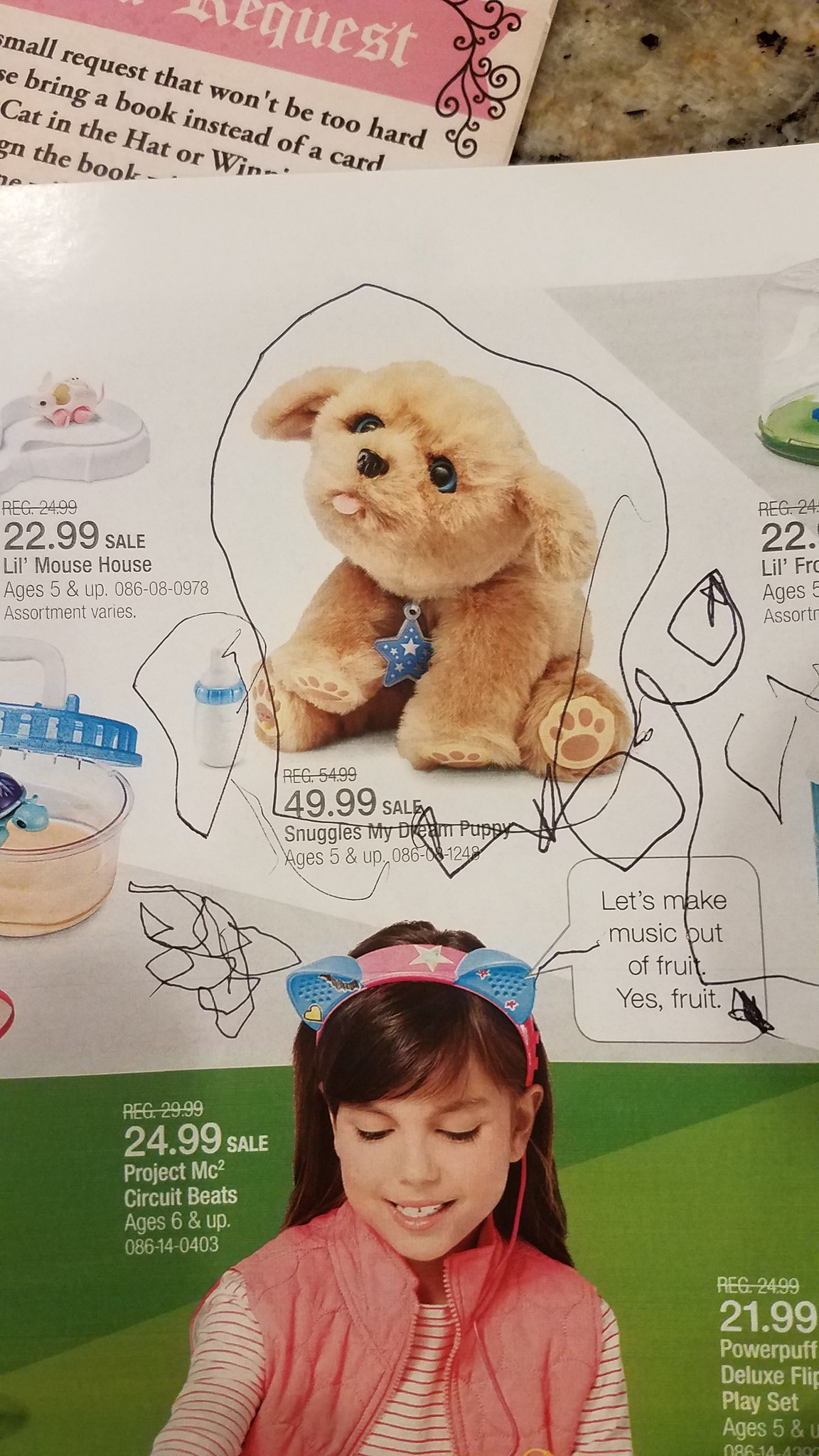This image is an extreme close-up of a cluttered tabletop entirely covered by papers, dominated by a colorful catalog page. The main feature on the catalog is a well-groomed plush doggie priced at $49.99, with its price circled and black scribbles reminiscent of a child’s doodles surrounding it. The plush doggie has soft brown fur, exaggerated paw print shapes, wears a blue star around its neck, and appears to be looking up at the camera while sticking out its pink tongue. Below the plush doggie, there's a photograph of a young girl with long brown hair, wearing a pink headband with blue cat ears, a pink jacket vest, and a white and pink striped shirt. Next to her image is a price tag of $24.99. The catalog also features text bubbles, one of which reads, "Let's make music out of fruit, yes fruit," suggesting it might belong to a toy advertisement for kids. At the bottom edge of the image, partially obscured by the catalog page, there’s another piece of paper mentioning a small request about bringing a book instead of a card. The image conveys a playful and somewhat chaotic snapshot, possibly invoking a child’s energetic interaction with the catalog.